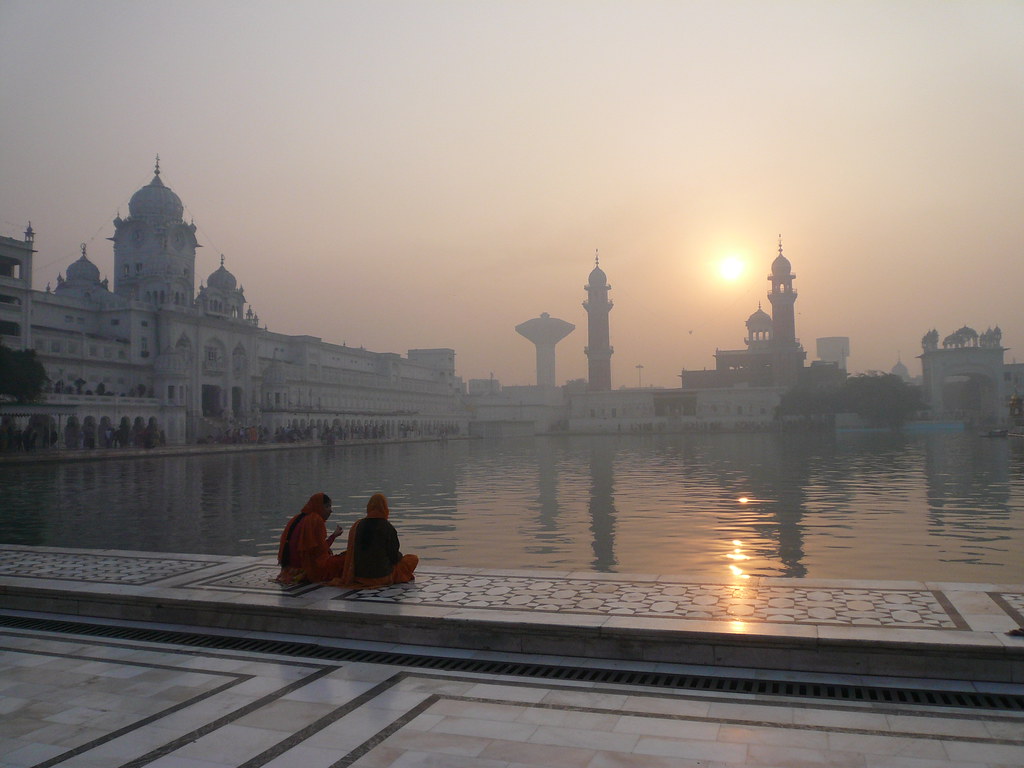In the image, two individuals wearing red burqas sit side by side on what appears to be a wide, paved marble bench, overlooking a massive, square-shaped waterway. The burqas cover their entire bodies, including their faces and heads, lending them an air of anonymity as they observe their surroundings. The expansive area around them is paved with marble blocks, contributing to the serene and grandiose setting.

Stretching in front of them and curving around the waterway is a vast, majestic temple characterized by multiple domes and arched entryways, with several towering minarets piercing the hazy sky. The architectural marvel creates an almost ethereal backdrop with numerous windows and intricately designed archways, some adorned with statues.

The environment seems to be shrouded in a misty haze, possibly due to a sandstorm or heavy smog, filtering the low, afternoon sunlight into a muted glow. This diffused light softly reflects off the tranquil surface of the water. Very little greenery interrupts the scene, with only a few trees and bushes sparsely scattered across the marble landscape. The overall composition evokes a sense of quiet reflection and timeless beauty amidst an architecturally rich and spiritually significant setting.